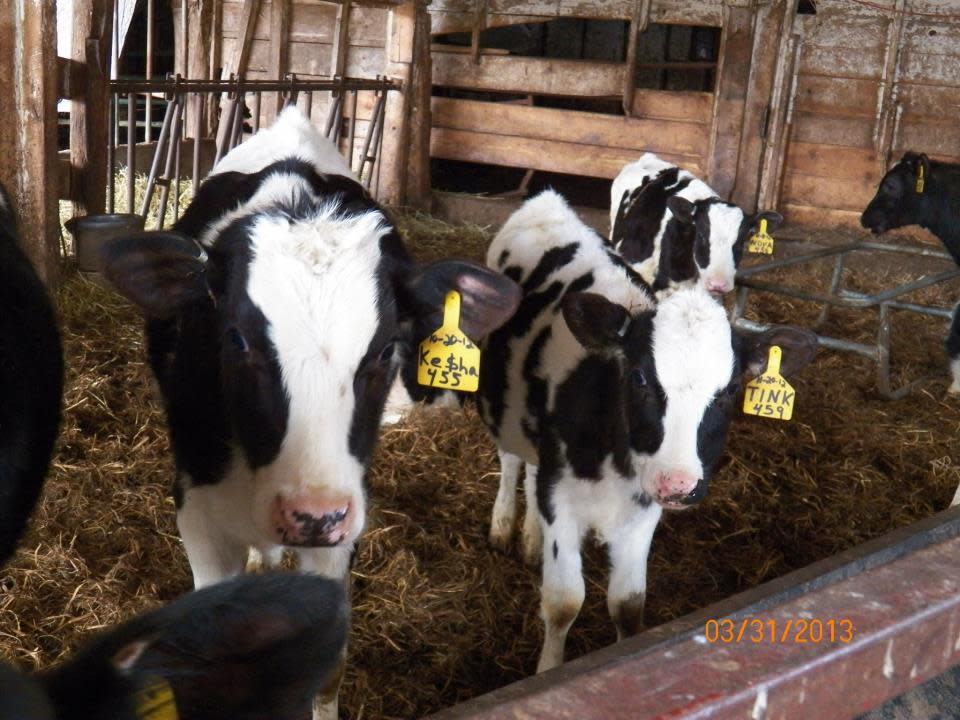A vibrant, sunlit image captures the scene of five cows in a pen, with the three most prominent cows standing on a bed of hay. Each cow sports a yellow ear tag adorned with details in black ink. The closest cow’s tag reads "Keisha" with a stylized dollar sign for the 'S,' her number being 455, and the date 10-20-12 (October 20, 2012). The middle cow has a tag that reads "Tink 459," dated 10-26-12 (October 26, 2012). The tag of the far-right cow is not legible. A wooden board spans the background, adding a rustic element to the setting. Sunlight streams in from the upper right, illuminating the pen warmly. In the lower right corner of the image, an orange digital timestamp marks the date 03-31-2013, indicating the photograph was taken on March 31, 2013.